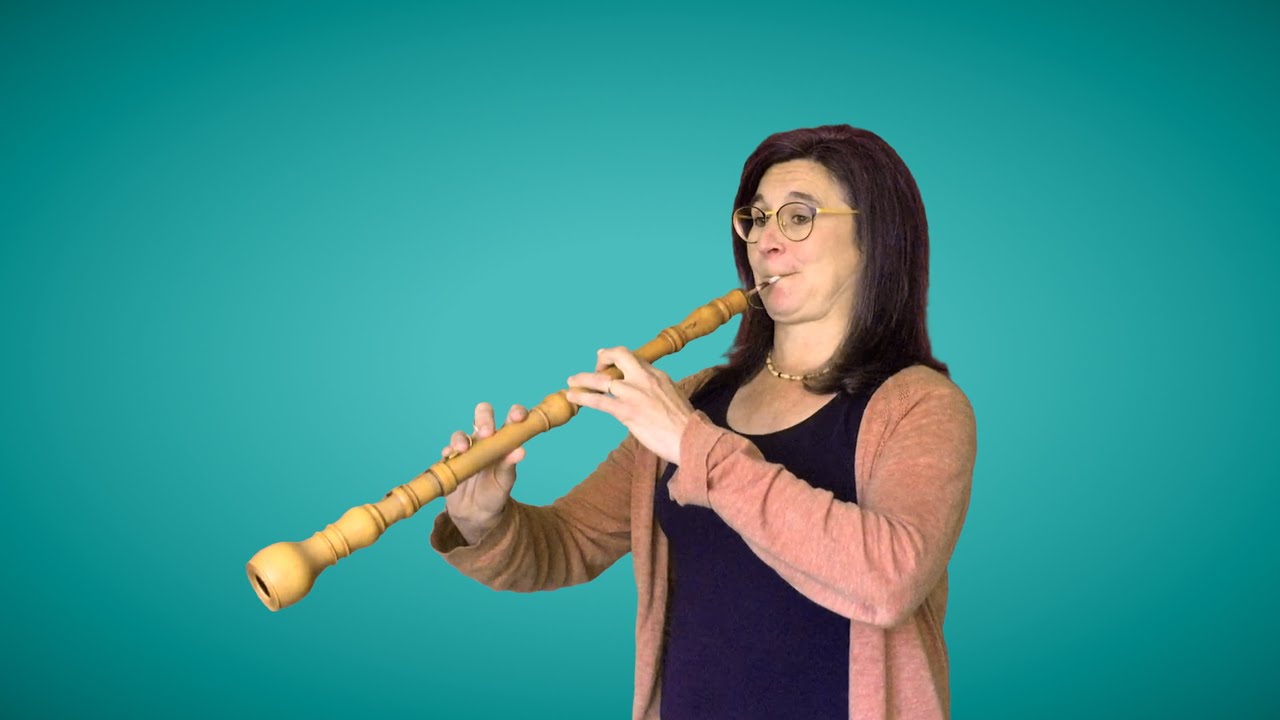The image depicts a woman deeply engaged in playing a wooden, elongated woodwind instrument resembling a clarinet. Her dark brown hair, interspersed with gray strands, cascades around her face as she focuses intently on the instrument. She wears distinctive glasses with gold ear handles and blue rings, which frame her eyes clearly. A black shirt with a half-circle neckline is layered with a vibrant, red coral shawl-like drape featuring long sleeves. Underneath, she sports a purple t-shirt. A ring adorns the second finger of her left hand, which grips the instrument near the top, while her right hand steadies it near the bottom at a 45-degree angle. Her cheeks are puffed, emphasizing her effort in playing, while her slightly raised eyebrows hint at her concentration. In the background, a teal gradient shifts from a brighter center to darker edges, providing a vivid contrast to her figure.